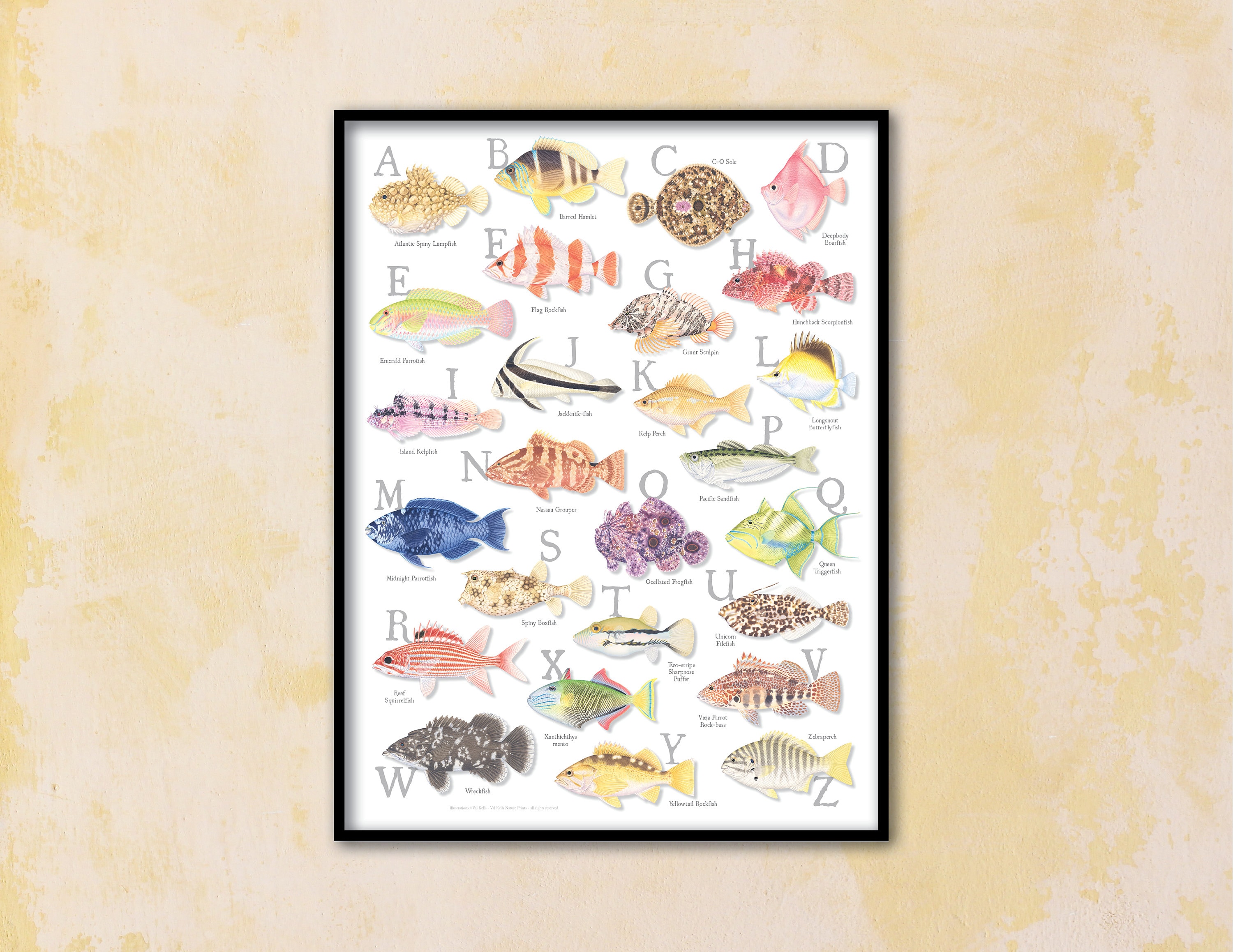The image depicts a framed educational poster of various fish species, arranged alphabetically from A to Z. The poster itself features a diverse array of fish, each distinctly colored, and labeled with both their common names and corresponding letters of the alphabet. The background wall is primarily a peachy tone with light orange splotches, giving it a textured appearance, which accentuates the black-bordered frame of the poster.

Each fish is meticulously illustrated with vibrant colors ranging from blues, reds, purples, and yellows to browns and greens. The A fish, an Atlantic spiny lampfish, is brown, while the B fish is a brown and white striped species with yellow fins and a white tail. Notable other species include the yellow-tailed, brown-striped zebra perch (Z) and the queen triggerfish (Q), which blends green and blue shades. The entire depiction serves both as an informative piece and as an artistic showcase, making it ideal for educational purposes and visually captivating as wall decor.